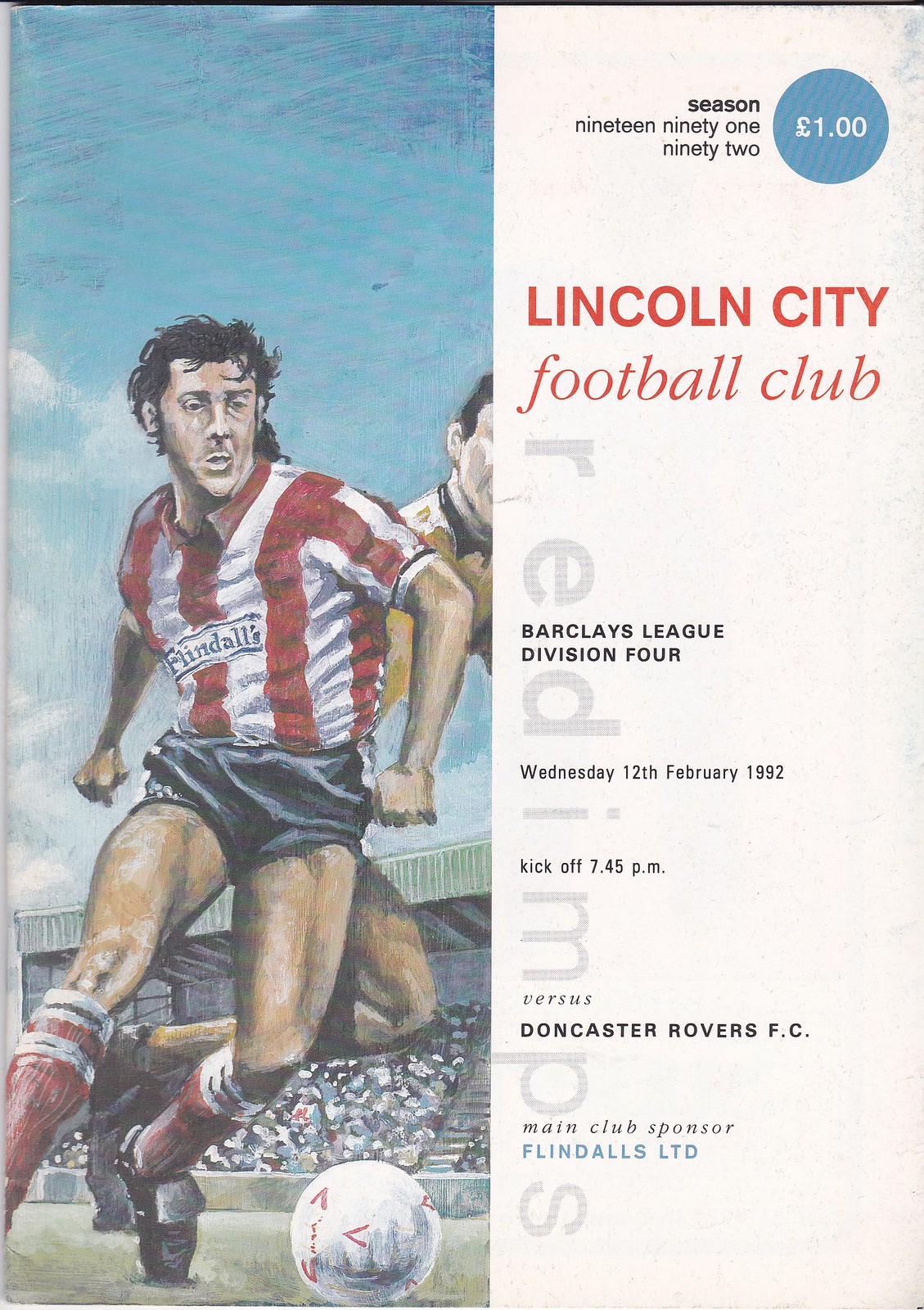The cover of this contemporary game day magazine for Lincoln City Football Club, season 1991-92, is divided into two sections. The left half features an illustration of a soccer player in action, donning a red and white vertically striped jersey with a sponsor's name across the chest, blue shorts, and red socks with white stripes at the top. He's skillfully dribbling the ball down the field, pursued by a defender in a yellow jersey, with a grandstand full of enthusiastic fans in the background.

On the right side of the cover, a white background hosts several pieces of text information. At the top, it reads "Season 1991-92" in large, clear text next to a price of 1.00 in a denomination (L or €). Below, in red and black text, it states "Lincoln City Football Club." Further down, the details of the match read: "Barclays League Division 4, Wednesday 12 February 1992, Kickoff 7:45 PM, vs Doncaster Rovers FC." The main club sponsor, "Flindalls Ltd," is mentioned at the bottom.